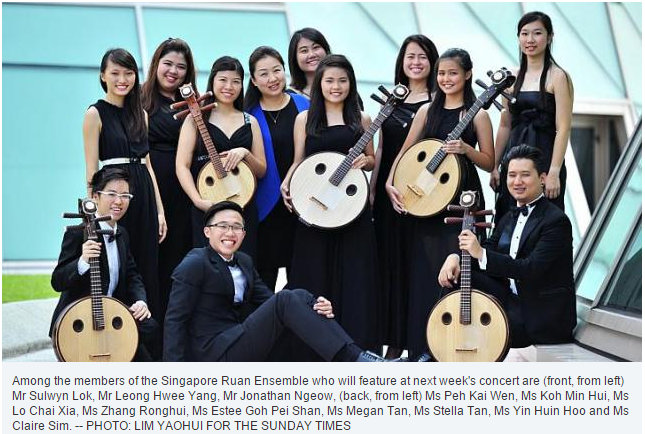In this horizontally oriented photograph, the members of the Singapore Ruan Ensemble are gathered in front of a modern building with large glass windows. The group, composed of individuals of apparent Asian descent, includes ten women and three men, all formally dressed in black. The men are in dark suits and bow ties, while the women wear a variety of black dresses, some with straps, others strapless or halter-topped.

The ensemble members are arranged with three men seated in the front and ten women standing behind. Positioned centrally among them is a woman distinguished by a blue sweater or wrap over her black dress. All are smiling at the camera. Each of the five musicians holding instruments are wielding traditional round stringed instruments similar in appearance to large banjos, with face-like holes on either side of the bridge and long necks.

The caption below the image identifies the ensemble members: "Among the members of the Singapore Ruan Ensemble, who will feature at next week's concert, are, front from left, Mr. Sulwin Lok, Mr. Leong Hui Yang, Mr. Jonathan Ngau, and back from left, Ms. Pei Kai Nguyen, Ms. Kho Nguyen Huy, Ms. Lo Chai Zai, Ms. Zeng Rong Hui, Ms. Estay Goh Pai Shan, Ms. Megan Tan, Ms. Stella Tan, Ms. Yin Huynh Hu, and Ms. Claire Sim." This image was captioned and published in the Sunday Times, photo credit to Lim Yahui.